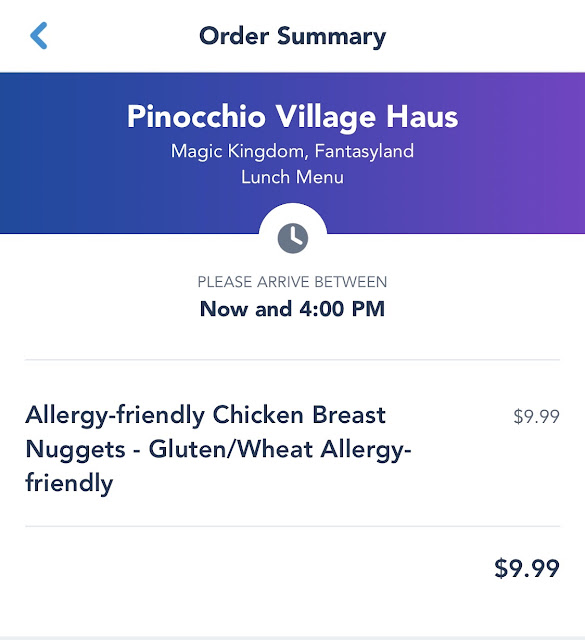This photo captures an order summary page from a mobile app interface. Prominently displayed at the top center is the title "Order Summary." In the upper left corner, there is an aqua blue back arrow, allowing the user to navigate to the previous page. Below this, there is a small gap followed by a rectangular banner that spans the width of the screen. This banner transitions from blue to purple and features white text in the center.

The text on the banner indicates the dining location, "Pinocchio Village Haus," situated in the "Magic Kingdom, Fantasyland." Below this, additional white text specifies the "Lunch Menu." The eye is drawn to a circular cutout in the center of the banner, which contains a silhouette of a clock. Underneath the clock, a message reads, "Please arrive between now and 4 PM."

Directly below this banner, the menu item is listed: "Allergy-Friendly Chicken Breasts Nuggets (Gluten/Wheat Allergy-Friendly)," priced at $9.99.